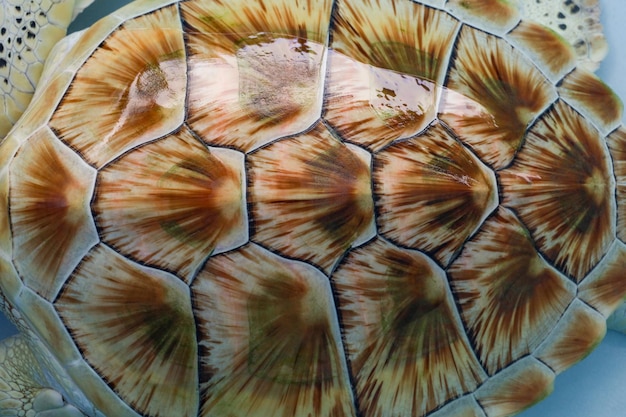This close-up image beautifully captures the intricate details of a turtle shell, likely belonging to a sea turtle or tortoise. The shell is oval-shaped and displays a glossy, reflective surface that highlights its natural beauty. Dominated by brown and orange hues, the shell features approximately 12 or more sections, each outlined in white with hints of black. The middle sections are smaller and similarly shaped, while the outer sections are larger and wider, contributing to a broken, almost pie crust-like pattern. Each plate on the shell carries a unique, flower-like design, adding to the shell’s aesthetic appeal. The image is zoomed in, revealing just the edges of the turtle's flippers, which are adorned with black spots on a yellow background. The shell's light brown ridge runs along the outer edge, framing the detailed patterns within. Although the image isn't professionally taken, it effectively centers the turtle shell, making its vibrant colors and textures the focal point. There is a hint that the turtle might be inside the shell, as evidenced by light scales visible at the corners of the image.